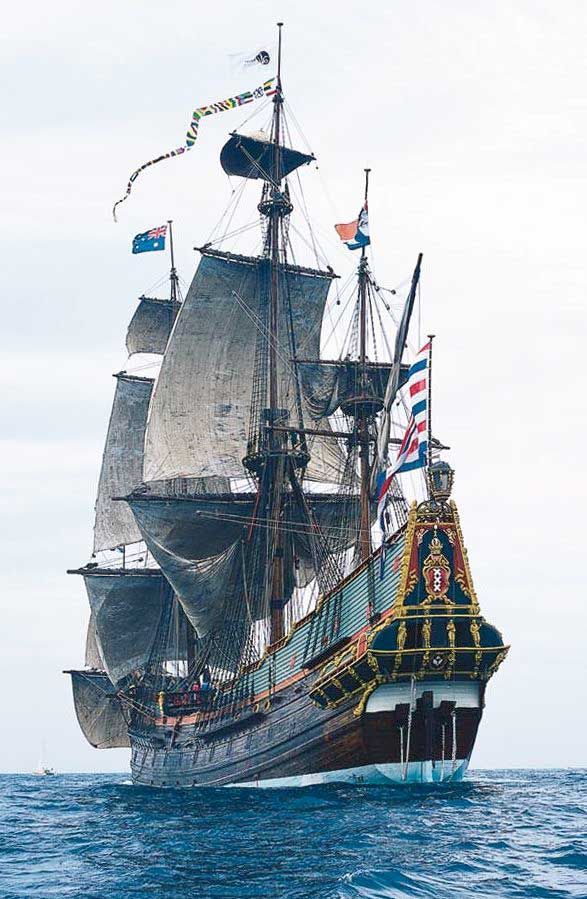This is a color photo of an immense, vertically rectangular wooden ship on the open sea. The ship, likely refurbished and elaborately ornate, has a Victorian style with dark blues, reds, and crowned golden symbolism. Its three masts prominently display several flags: the New Zealand flag on the first mast, a strip of semaphore flags below a white flag with black markings on the middle mast, and a partly furled flag with white, red, and blue alternating stripes on the rear mast. The deck is enclosed, giving it a posh, extravagant appearance, reminiscent of a Victorian household. The image, taken from water level looking up, reveals numerous tie lines and ropes that connect the deck to the sails above, which are currently open. The front of the ship bears three letters, "XXX," and there is an identifiable Great Britain flag in the upper left. The background showcases a light sky, predominantly white with faint clouds and a hint of blue, while the sea appears blue with gentle movement. The photograph, slightly grainy, captures a serene yet majestic maritime scene.